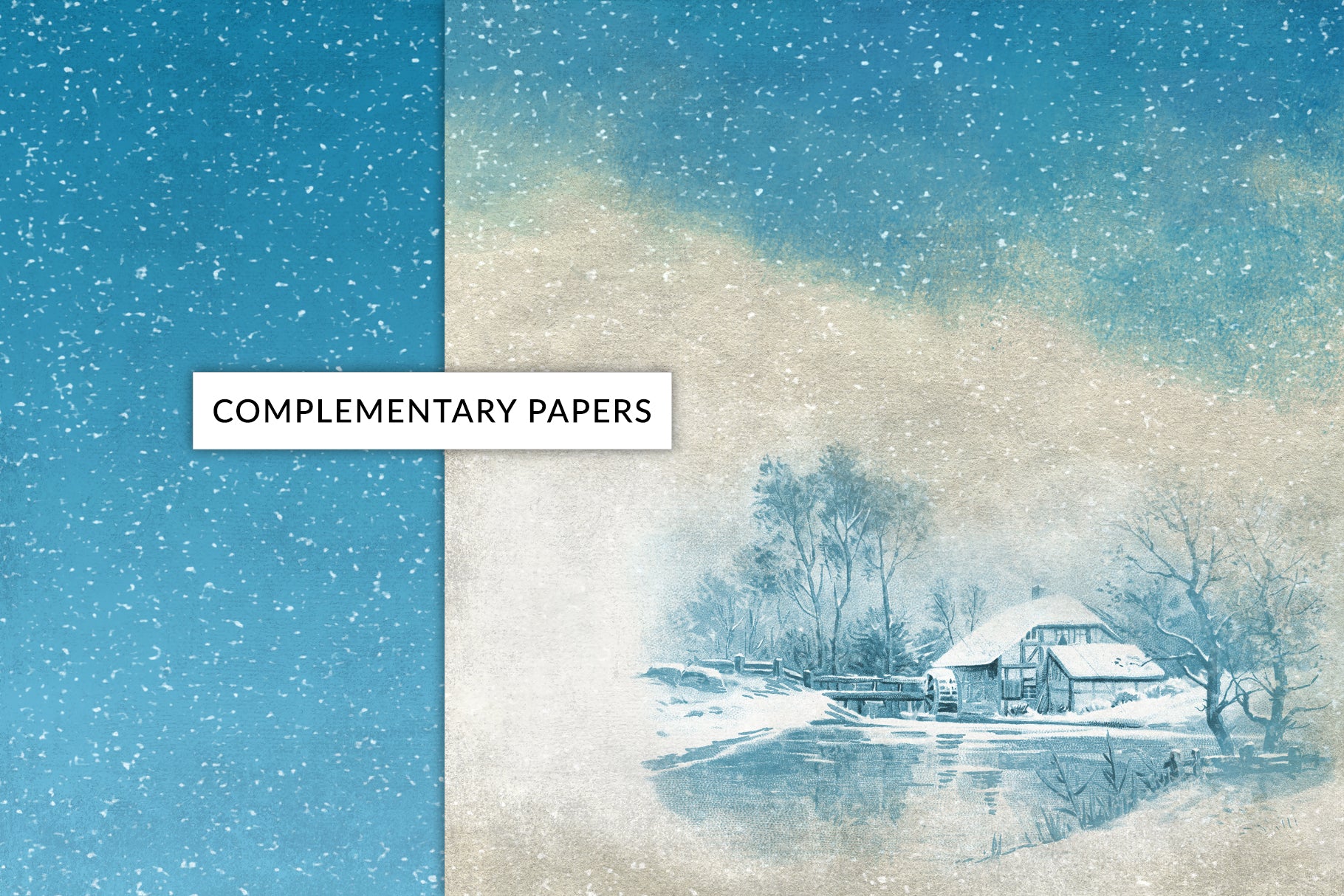The image is a detailed color illustration with elements of graphic design, reminiscent of a Christmas card. It features a picturesque winter scene, dominated by a snowy house with a waterwheel, likely a mill, situated beside a river that may be partially frozen. The scene exudes a heavy snowfall feel, with bare trees and accumulating snow on the ground, roof, and waterwheel. The sky above is a deep aqua-blue, dotted with white snowflakes or stars, blending seamlessly from a white-beige cloud effect into the blue sky, covering about three-fourths of the right-hand side. The left side is a solid blue with white star-like images, creating a cohesive theme across the illustration. This wintery scene is framed within a horizontal rectangular layout, and the left-hand side prominently features a white block font reading "complementary papers." The style merges traditional illustration techniques with modern graphic design elements, producing a nostalgic yet contemporary visual experience.